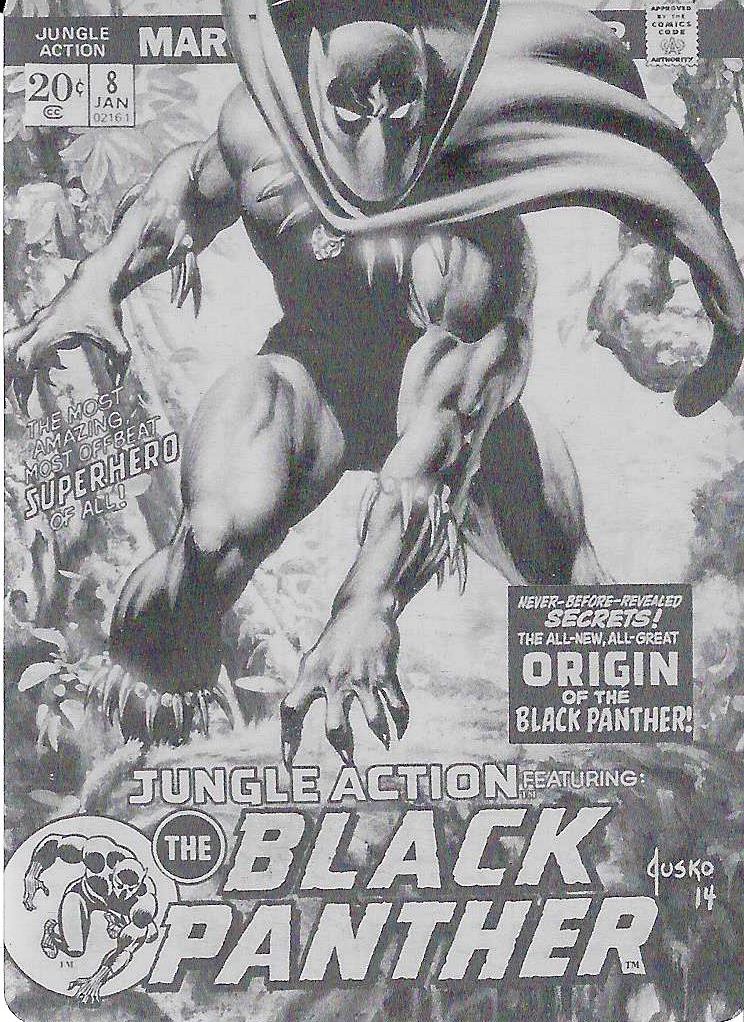This black-and-white comic book cover features "Jungle Action" with the Black Panther, showcasing its vintage nature with a price of just 20 cents. At the top, a partially obscured "MAR" banner is visible. Central to the cover is an image of the Black Panther in a dynamic pose, with claws extended and cape billowing, giving the impression that he is leaping towards the viewer. A text box on the left declares, "The most amazing, most offbeat superhero of all!" Below this main figure, another text box proclaims, "Never before revealed secrets, the all-new, all-great origin of the Black Panther." The issue is dated "8 Jan" and is marked as number 14 with a specific code "02161," possibly indicating the year 1961. Additionally, the bottom of the cover reads, "Jungle Action featuring the Black Panther." A Comics Corp. approval stamp is located in the upper right corner, and an emblem of the Black Panther appears in a circle at the bottom left, reinforcing the iconic status of this classic superhero.